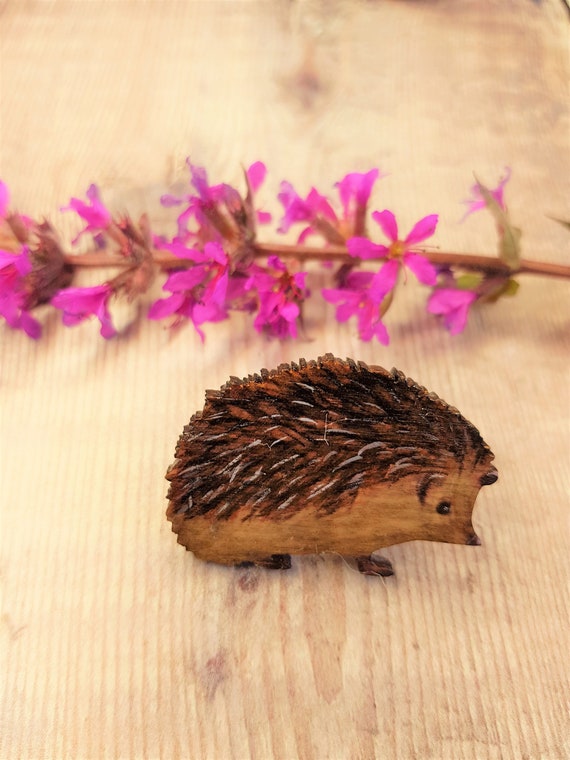This is a vertical photograph featuring an intricately carved wooden hedgehog placed on a light-colored wooden table, showcasing its grain. The hedgehog, meticulously crafted with fine details, including its spines, small feet, eyes, pointy nose, and ears, sits on top of a larger piece of wood. The carving of the hedgehog’s spines demonstrates impressive craftsmanship, appearing almost like fur. Behind the hedgehog is a single brown sprig adorned with multiple fuchsia pink flowers, each boasting five petals and a small yellow center. The sprig, lying horizontally across the image, adds a vibrant contrast against the detailed wooden artwork, creating a harmonious blend of natural elements and artistic skill. The overall composition captures the essence of detailed craftsmanship and natural beauty.